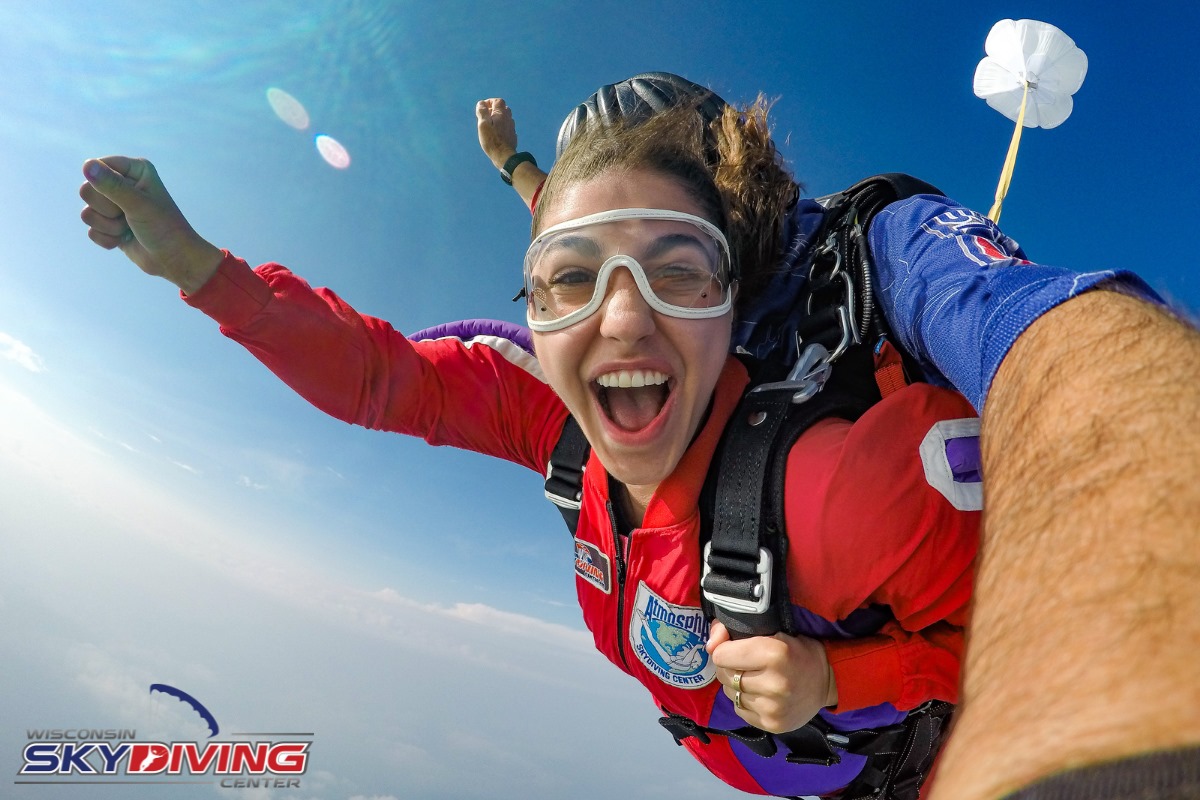The image captures the exhilarating moment of two skydivers in mid-dive, framed in a landscape-oriented, color photograph taken with a GoPro camera. In the foreground, a woman wearing white goggles and a red jumpsuit with a black harness is pictured, her mouth open in a joyous yell and her right fist triumphantly raised. Above her, a man in a blue jumpsuit, presumably her instructor, has his arm securely wrapped around her for guidance. His left fist also mirrors the woman's pose, raised in the air. The backdrop of a clear blue sky and some clouds adds to the sense of height and adventure. A partially deployed white parachute hovers above them to the upper right, signaling that their descent is carefully controlled. In the lower-left corner, the image is branded with the Wisconsin Skydiving Center logo, adding a professional touch to this thrilling scene.